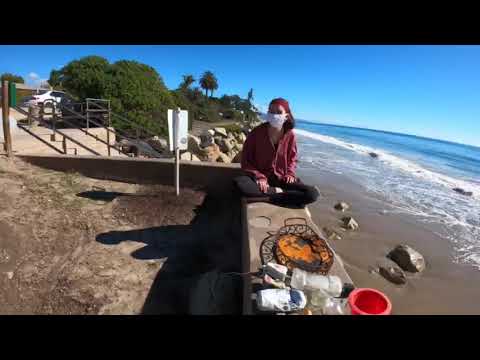The image captures a serene, yet somewhat cluttered scene at the beach, featuring a woman with red hair who is seated comfortably in an Indian style position on a concrete beach wall. She is wearing a red blouse, black pants, and a white face mask, appearing to be either setting up or organizing an assortment of items in front of her, including what might be cookware and a basket with an orange substance. Spread out neatly before her is a collection of empty, crushed bottles and other pieces of trash, seemingly arranged for a purpose. The setting extends to the right where wet sand slopes gently down to the ocean, and a stone staircase leads from the beach up a small hill dotted with dirt, large bushes, and small trees. Additionally, the scene is segmented by two long horizontal black lines at the top and bottom. In the upper left, a white car is parked under a blue sky mixed with some white clouds.